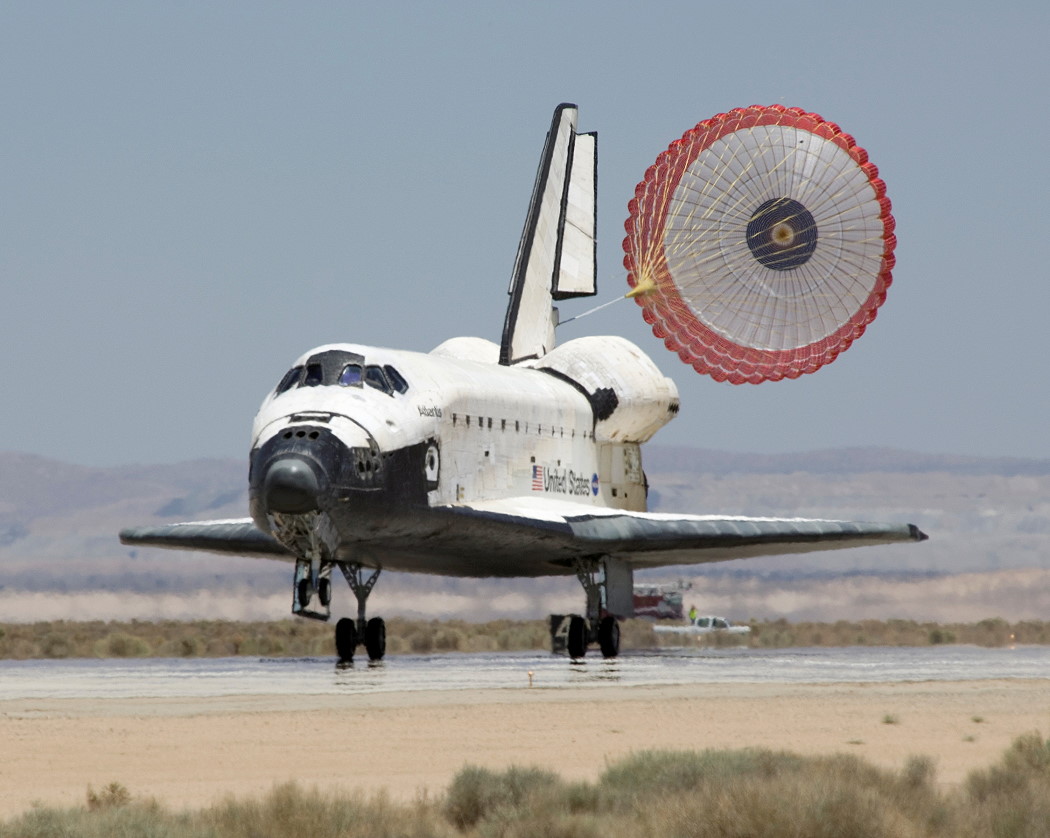In this detailed image, a United States Space Shuttle is captured landing on a desert runway. The Space Shuttle, characterized by its white upper body and black underside, prominently features a United States flag, the words "United States," and a NASA logo on its side. The scene is viewed from a side angle, showing the Space Shuttle decelerating with the assistance of a large parachute that has red, white, and black sections. The shuttle's landing gear is fully deployed, with the main body wheels touching down on the runway, while the front nose landing gear is still slightly airborne as it prepares to make contact.

The setting is a desert environment with greenish, dark brown, and grayish desert vegetation visible both in the foreground and background. You can also spot scattered scrub brush and tumbleweeds along the runway. In the distant background, small mountains rise against a grayish-blue sky. Additionally, a white pickup truck is seen far off in the distance, adding to the sense of scale and remoteness in this rugged landscape. The photograph offers a clear, professional view emphasizing the technical details of the spacecraft and the stark desert setting of its landing.